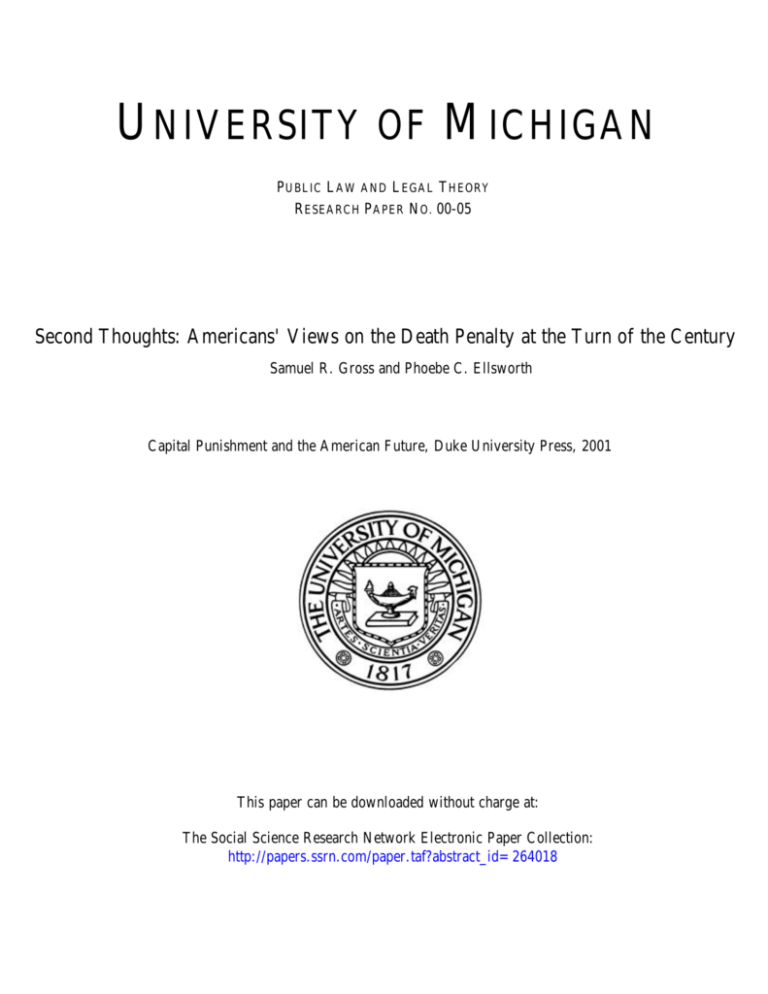**University of Michigan Paper Cover**

The cover page of the research paper features a clean, white background. At the top center, bolded black sans-serif text reads “University of Michigan,” with the 'U' and 'M' distinctly highlighted in bold. Directly below, smaller gray text in all capital letters announces “PUBLIC LAW AND LEGAL THEORY,” followed by “RESEARCH PAPER NUMBER 00-05” on the next line.

Further down the page, after some white space, the title appears in standard black text: “Second Thoughts: Americans' Views on the Death Penalty at the Turn of the Century.” Below the title, smaller text lists the authors, “Samuel R. Gross and Phoebe C. Ellsworth.”

Continuing downward, after another section of white space, a similarly sized line of text notes the publication details: “CAPITAL PUNISHMENT AND THE AMERICAN FUTURE, Duke University Press 2001.”

Toward the bottom, the University of Michigan seal is prominently displayed. The seal features text curving from the bottom left quadrant to the bottom right, reading “The University of Michigan.” Within the seal, a shield displays an inscribed genie lamp image, all rendered in a black ink style. At the bottom of the seal, the year “1817” is inscribed.

Finally, at the bottom of the page, text mentions, “This paper can be downloaded without charge at the Social Science Research Network Electronic Paper Collection.” Beneath this sentence, the URL is presented in blue text: [http://papers.ssrn.com/paper.taf?abstract_id=264018](http://papers.ssrn.com/paper.taf?abstract_id=264018).